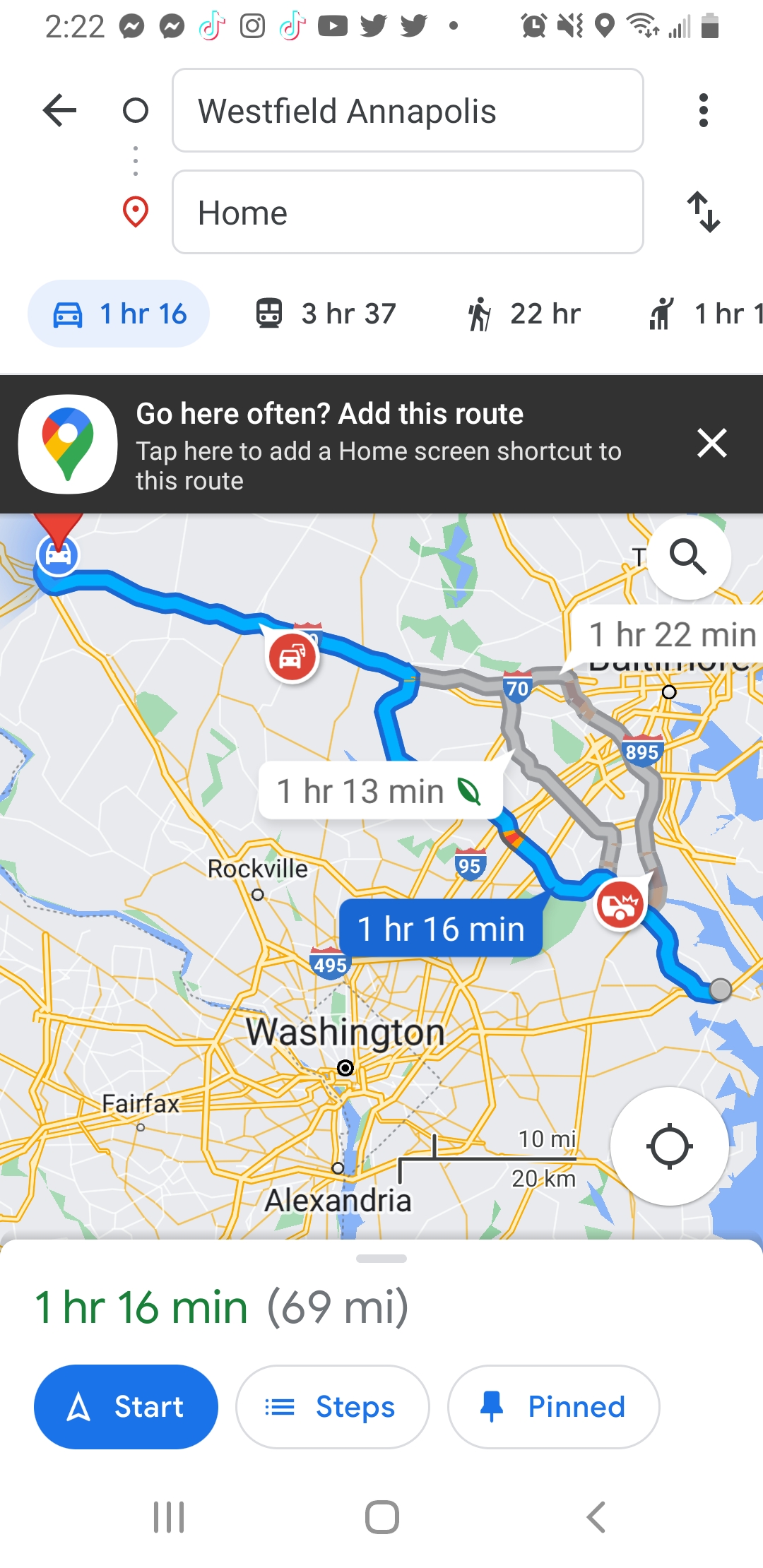This image is a detailed screenshot of Google Maps on a mobile phone. The top of the screen features the typical status bar with various icons indicating the Wi-Fi signal and app notifications including Twitter, YouTube, Instagram, and Messenger. Below that, the interface shows "Westfield Annapolis" in black text on the top bar and "home" in black text on the bottom bar, suggesting the user is looking to navigate from Westfield Annapolis back home. 

The central area of the screenshot displays the map itself with a gray background and a blue line showing the selected route. Various transportation icons indicate the duration for each mode of travel: a car (1 hour 16 minutes), a train (3 hours 37 minutes), walking (22 hours), and possibly an Uber option partially visible. At the bottom, another white bar contains green text stating "1 hour 16 min" and gray text in parentheses showing "69 MI." Three ovals at the bottom serve as action buttons; the one on the left is blue with white text "Start" and a white arrow outline.